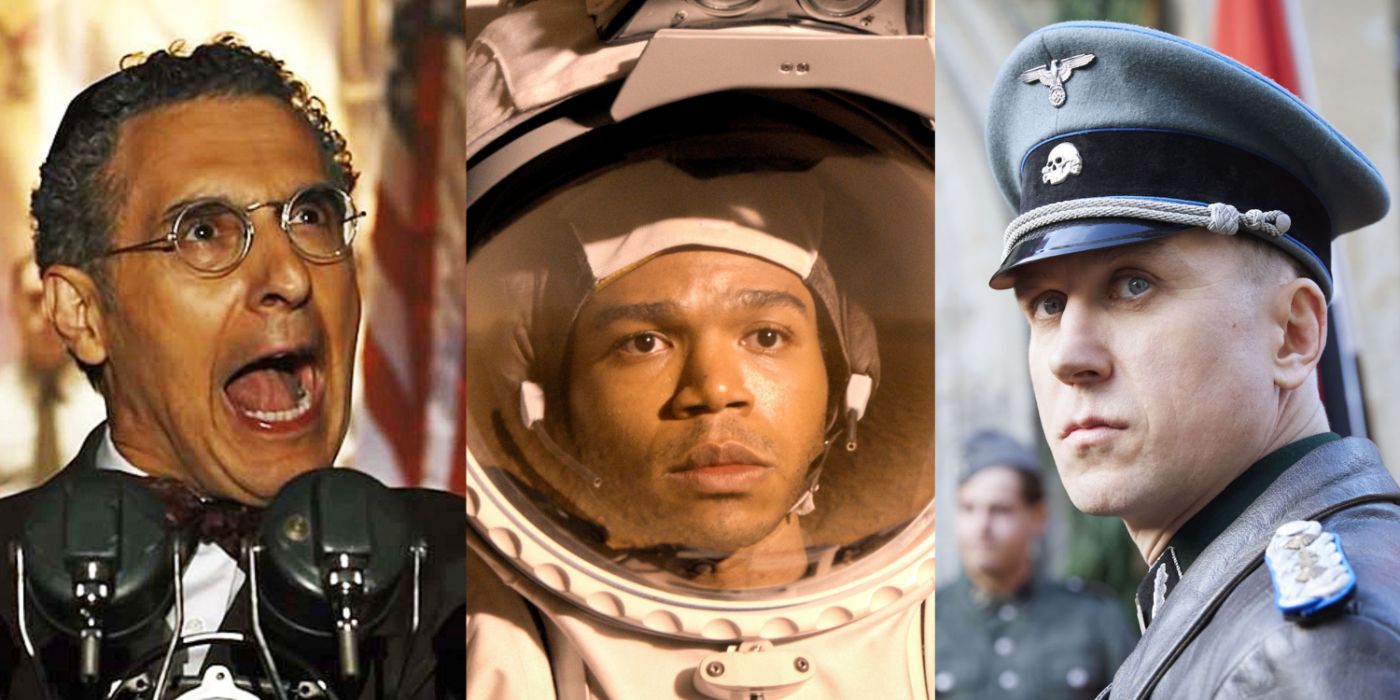The image consists of three individual headshots aligned from left to right, each capturing a different scene and persona. On the left, a man with wire-rimmed round glasses and short, slicked-back black hair, likely in his 50s, is shouting passionately into two vintage microphones. He is dressed in a black suit, white shirt, and bow tie, with an American flag visible behind him. The middle photograph features a serious African American man wearing a white astronaut suit, with a sturdy helmet visible that reveals his face through the glass visor, staring intently ahead as if contemplating a significant moment or sight. The right-hand image shows a Caucasian man in a gray military uniform adorned with three or four stars on his shoulder, indicating a high rank, possibly a general. He wears a gray military hat with a black band and insignias including an eagle pin, and he looks solemnly over his shoulder with a hint of a red, green, and white flag in the background.